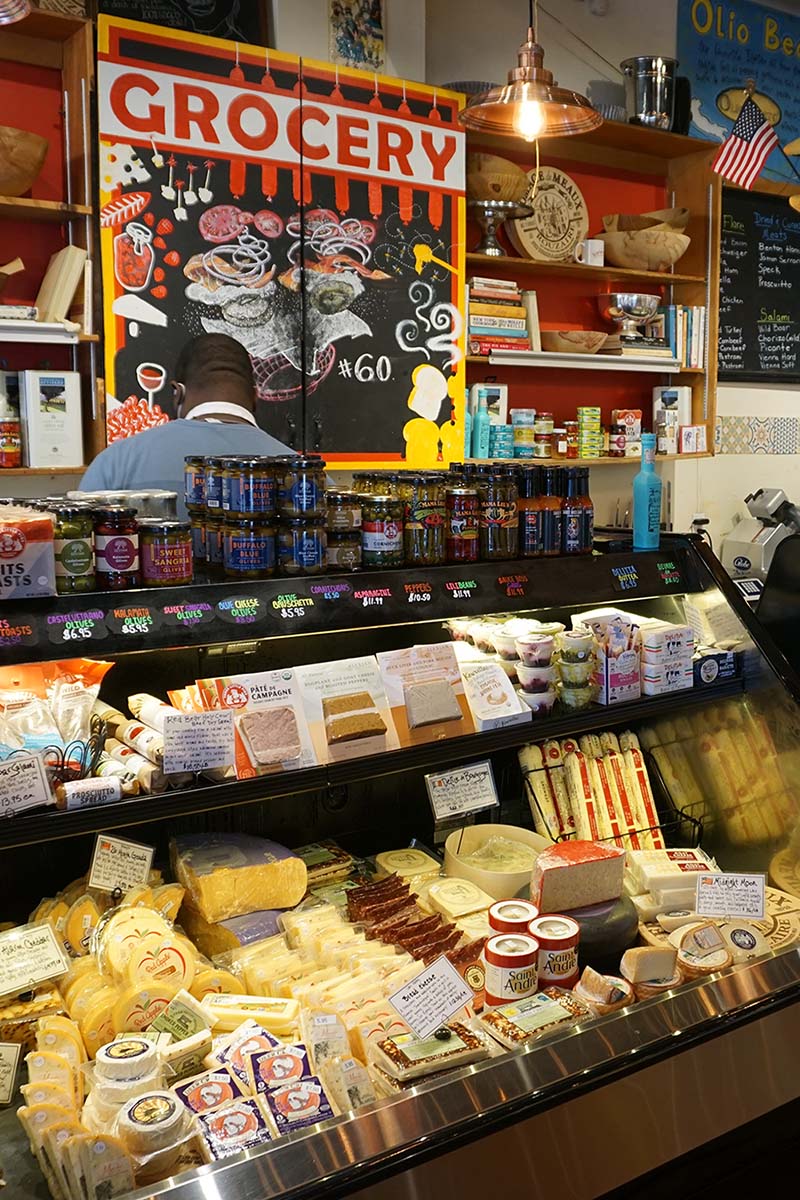The image captures the interior of a small, homey grocery store, focused on a deli section. Front and center is an open refrigerated case displaying a variety of cheeses on the bottom shelf, while the top shelf holds jars of pickles, cherries, olives, and small containers of spreads and dips. Behind the counter stands an African-American man, wearing an apron with the strap visible around his neck, busily at work and possibly wearing a mask. Over his shoulder, a large sign reads "GROCERY" with a decorative design and the hashtag #60. On the far right of the image, an American flag hangs on the wall, adding a patriotic touch, and a chalkboard with handwritten notes lends a personal, independent shop feel. The ceiling holds a subtly lit light fixture, completing the cozy ambiance of this well-detailed deli section.